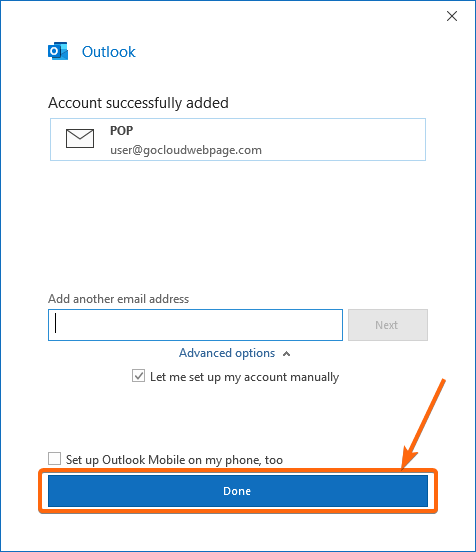This image features a successful addition of an Outlook account for the user "user@gocloudwebpage.com." The account information is displayed inside a square, marked by a distinct blue outline. Situated next to the email address is an envelope icon, while an 'X' icon is positioned in the top right corner of the square, indicating a close option.

Below this are further account setup options. A blue text box with a cursor invites the user to "Add another email address." The "Next" button is grayed out, showing no immediate action can be taken. Additionally, an advanced options dropdown is available, highlighted in blue, with the "Let me set up my account manually" checkbox selected.

To the right, another option, "Set up Outlook mobile on my phone too," is present but remains unchecked. At the bottom of the setup screen is a blue "Done" button. This button is emphasized by an orange border and an arrow pointing at it, directing the user's attention. The entire setup interface is displayed against a clean, white background.